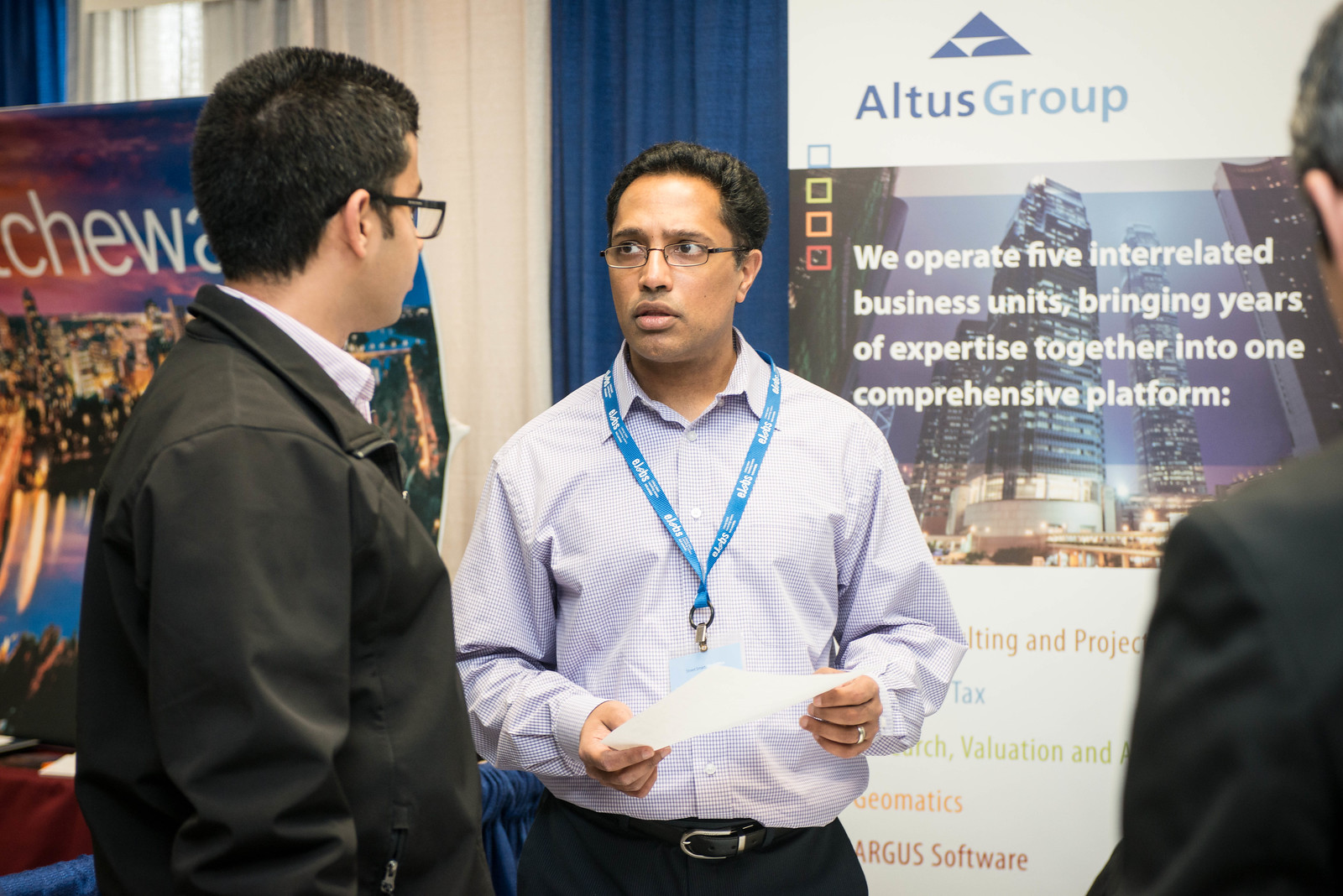In this indoor event photo, two gentlemen are engaged in conversation at what appears to be a trade show. Both men are wearing glasses. The gentleman on the left, with short black hair and lighter skin, is dressed in a black jacket over a white shirt, and looks to his right, engaged with the second gentleman. The man on the right has slightly darker skin and short black hair, and is wearing a light-colored, button-up shirt with a blue lanyard around his neck. He holds a piece of paper with both hands, and a ring is visible on his left hand. To the right edge of the image, a third person is partially visible from the shoulder up. Behind the central figures is a large banner for Altus Group, which reads, "We operate five interrelated business units, bringing years of expertise together into one comprehensive platform," with a city view depicted beneath the text. Blue and white curtains and additional posters are also visible in the background, contributing to the bustling trade show atmosphere.